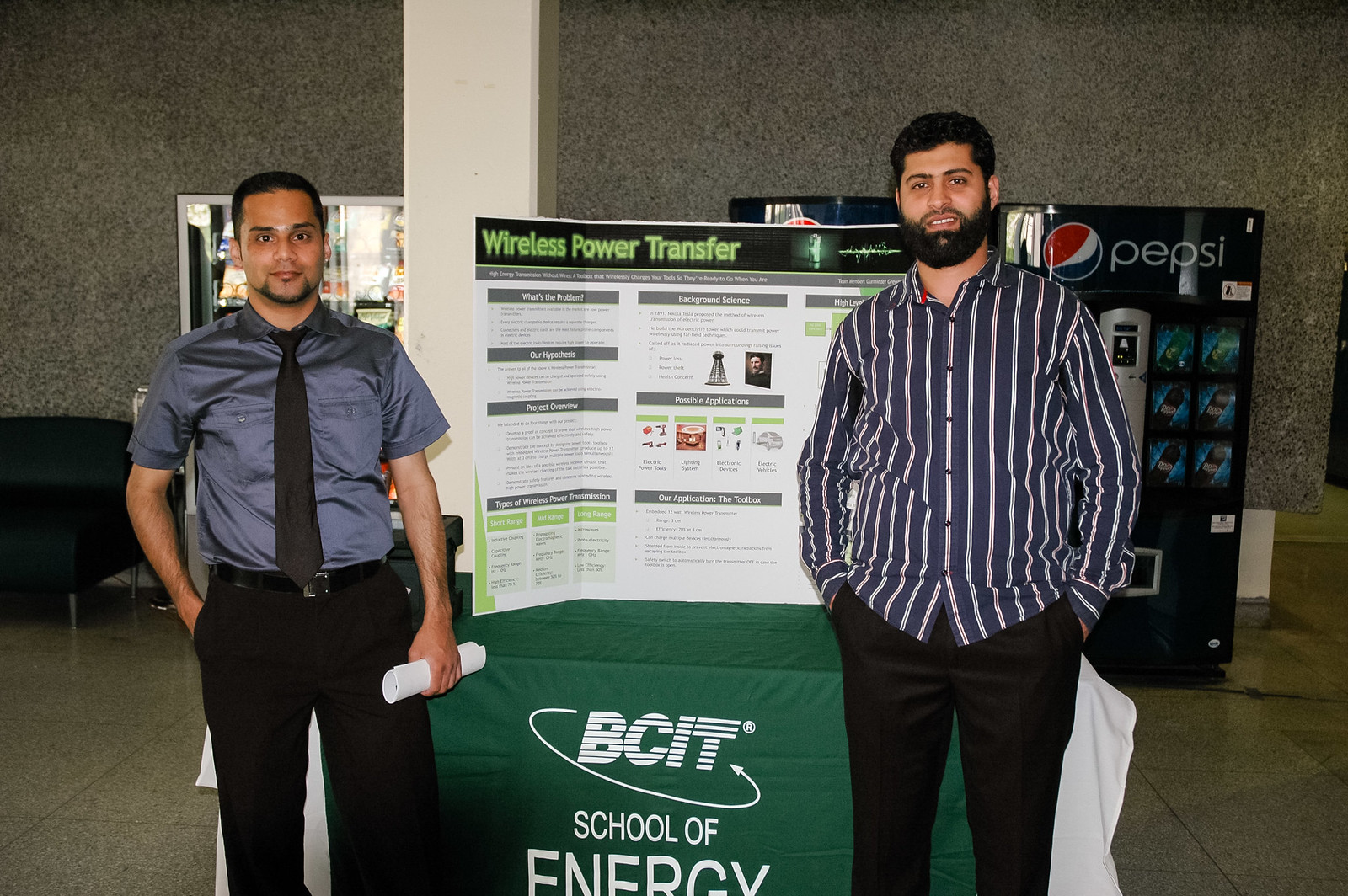The image depicts a presentation setup, likely at an educational or professional event, featuring two men standing in front of a detailed poster board. The poster prominently displays the title "BCIT School of Energy: Wireless Power Transfer" alongside various sections like "What's the problem," "Our hypothesis," "Project overview," "Background science," "Possible applications," "Our application," and "The toolbox," although much of the finer text is unreadable. 

At the center of the image is a table draped with a green and white tablecloth, also branded with "BCIT School of Energy." On the table rests the large poster board, which is white, gray, light green, and black. Two vending machines, a couch, and a pillar are also visible in the background, contributing dark blue, red, white, green, black, and gray tones to the scene. One vending machine features the word "Pepsi."

The man on the left has fair, caramel-colored skin, wears a blue short-sleeved button-down shirt with a black tie and black pants, and has a goatee and black hair. He holds a rolled-up piece of paper in his left hand. The man on the right, potentially of Middle Eastern descent, wears a blue and white vertical striped button-down shirt with black pants and sports a black beard. Both men stand in a large room with a marble wall in the background, setting a professional atmosphere for their presentation.